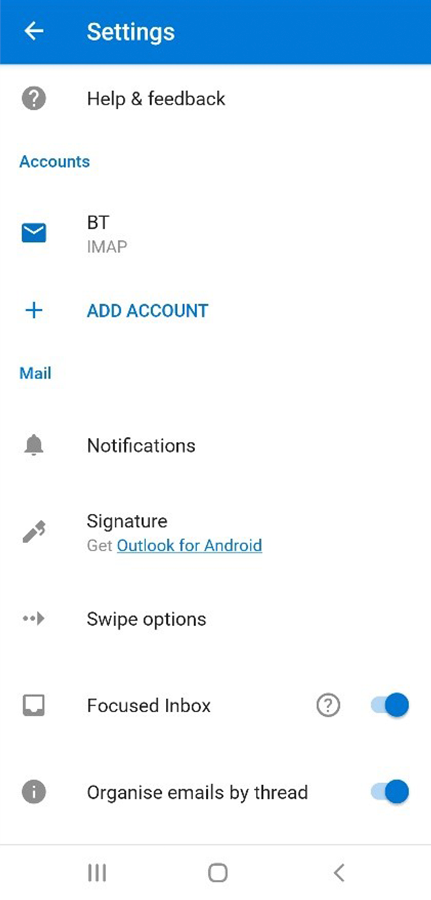A screenshot of a settings menu is displayed. The top of the screen features a wide blue bar with the word "Settings" in white text, alongside a back arrow on the left. Below this bar is a list of options, some of which are in grey and others in blue. The last two options have sliding switches beside them, both toggled to the right.

The options are listed as follows:

1. "Help and Feedback" in grey.
2. "Accounts" in grey.
3. "BTI map" in blue.
4. "Add account" in blue.
5. To the left of "Add account" it says "Mail" in blue.
6. "Notifications" in grey.
7. "Signature" in grey.
8. "Get Outlook for Android" in grey.
9. "Swipe Options" in grey.
10. "Focused Inbox" with the slider toggled to the right.
11. "Organise emails by thread" with the slider toggled to the right.

It is noted that "Organise" is spelled with an 's', which the observer points out as unusual compared to their customary spelling with a 'z'.